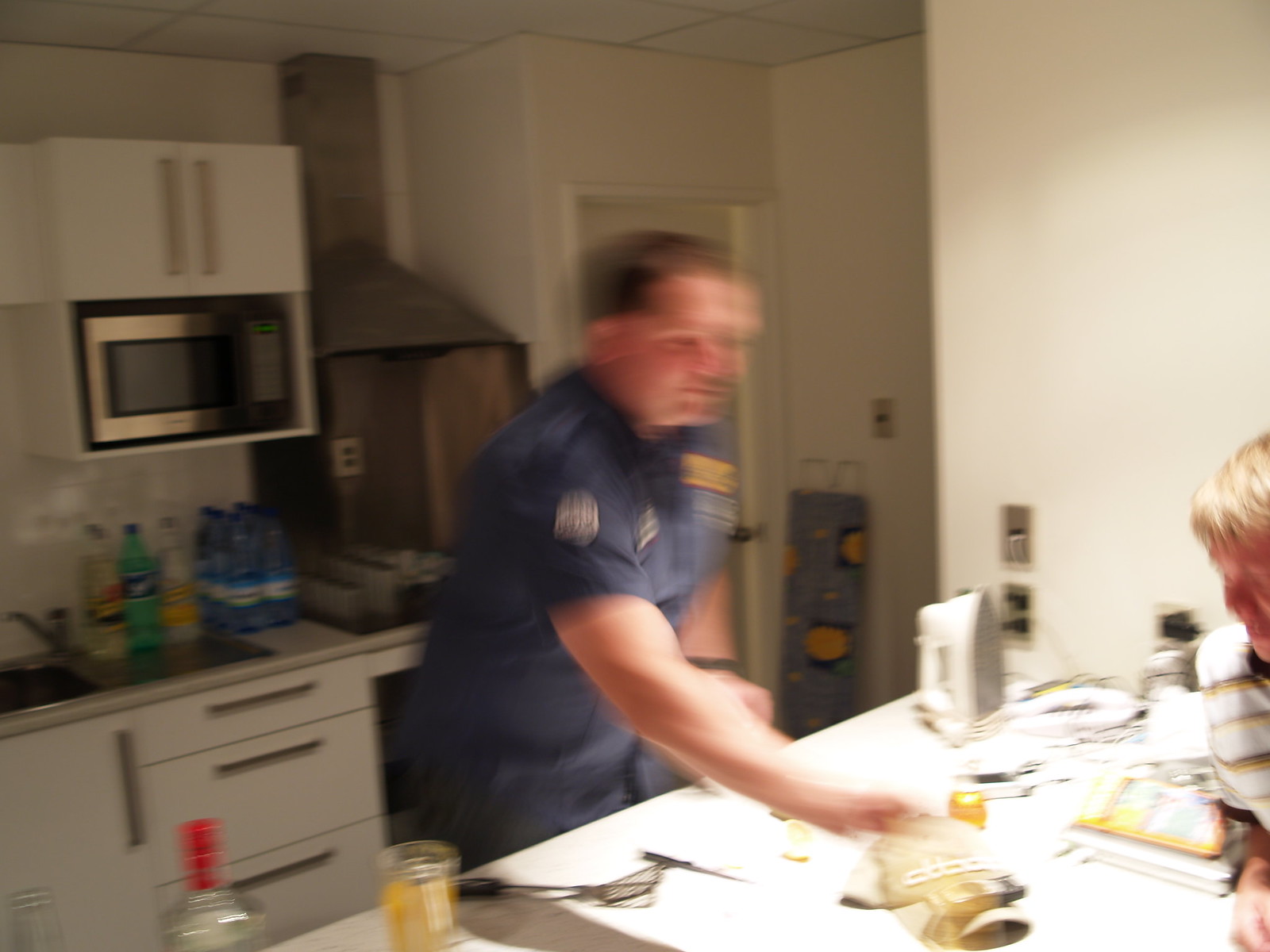In this rectangular photograph, a dimly lit kitchen scene is captured with the image appearing extremely blurred, reminiscent of double vision. The background features white walls adorned with silver-hardware cabinetry that houses a white microwave. To the right, there is what seems to be either a pantry door or an entrance to another room. Standing in the foreground, a man dressed in a dark gray uniform with a collared shirt and badges on both the upper arm and the front left chest is reaching over a white counter. On the counter, a white iron is prominently visible. From the right edge of the image, part of another person’s head emerges, displaying light-colored hair, either blonde or pale red, though their facial features are indistinct.